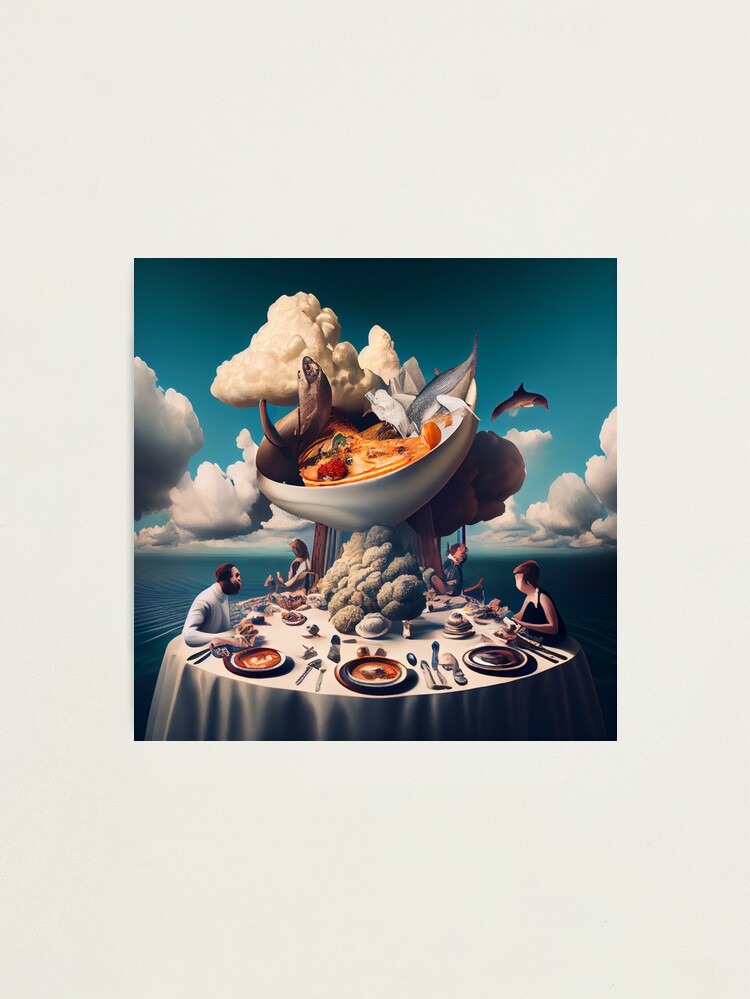In this surreal and detailed abstract artwork, an enchanting dining scene unfolds against a striking backdrop of a blue ocean and sky adorned with puffy white and off-white clouds. At the center of the composition, a large, round table bedecked with a pristine white tablecloth is set for approximately eight to nine guests. Plates, silverware, salt and pepper shakers are meticulously arranged on the table, which features an imposing, central centerpiece—a colossal bowl filled with sea creatures swimming in a mysterious yellow fluid.

Seated at the table are a formally dressed man with dark hair and a beard, donning a suit jacket, and a woman with dark brownish hair in a spaghetti strap black dress, their faces barely discernible. In the background, two more figures—another man and woman—stand, each turned away, mesmerized by the expansive seascape.

Adding to the magical essence of the scene, the sky above transitions from a deep blue-black hue at the top to a lighter blue closer to the horizon, framing the dreamlike tableau laid out below.